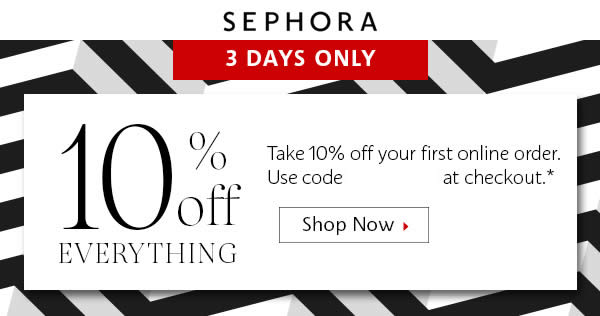The promotional image features a header with "Sephora" prominently displayed at the top. Directly below it is a red box with "Three Days Only" written in bold white text. The background of the entire design has a striking black zebra print pattern. 

Centrally located in the image is a large white box containing the main promotional message: "10% Off Everything." It further elaborates with, "Take 10% off your first online order. Use code," followed by a white-out section concealing the actual code text. The phrase "at checkout" is also included in this area.

Beneath this, there is a black rectangular box with the text "Shop Now" in white. Adjacent to this call-to-action is a small red arrow pointing to the right. The design aims to attract attention with its bold contrasts and clear, actionable instructions.